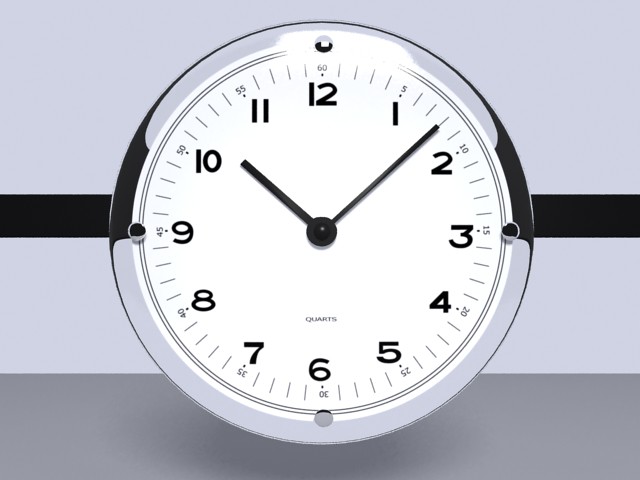The image depicts a detailed vector-style drawing of a thin-band watch with a prominent circular chrome frame around its white clock face. The clock, resembling one you might find in an office or school, features black numbers and hands. These numbers are conventional for a clock but include additional smaller numeric markers in increments of five, with the outermost ring displaying '5', '10', '15', and so on around the circumference, ending with '60' above the '12'. The current time is 10:08. The design is further accentuated with a shiny protective covering and a quintessential black horizontal bar in the background where the watch appears to hover a few centimeters above a tabletop. The overall background splits into horizontal sections, ranging from light grey at the top, a black horizontal stripe through the middle, and dark grey at the bottom. The word 'Quartz' identifies the clock's likely mechanism or brand.